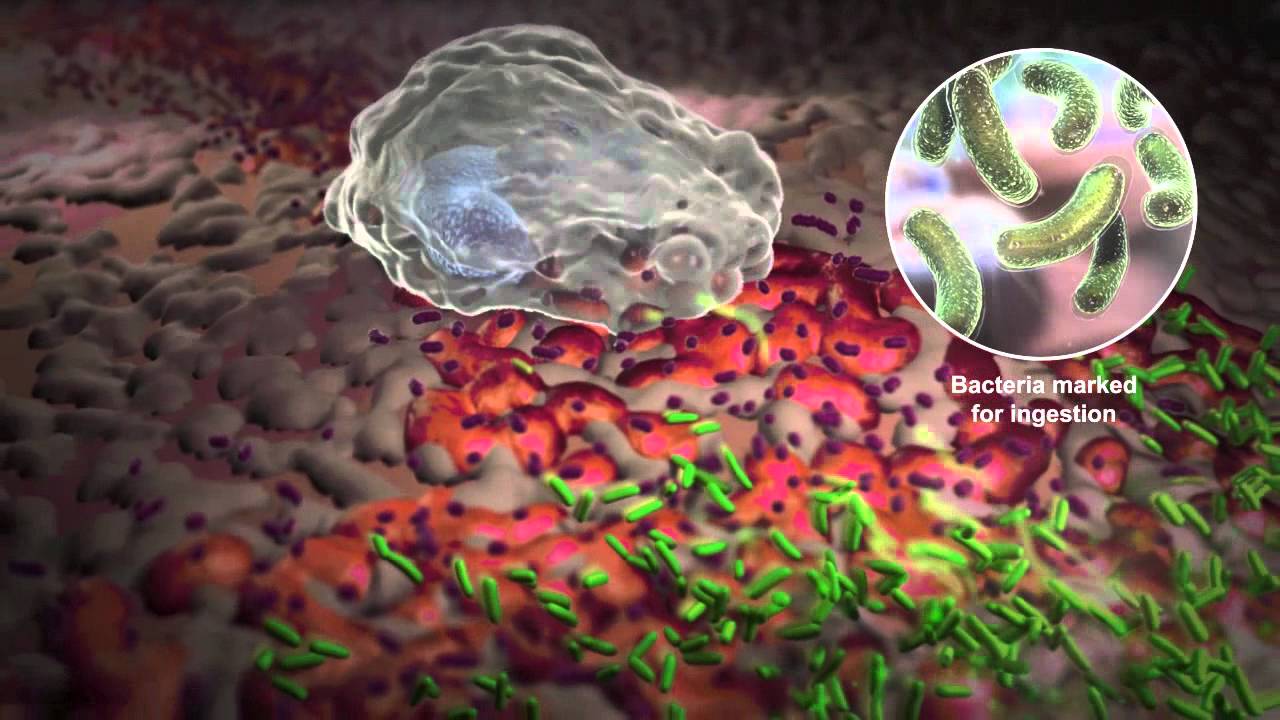The image is a detailed biological drawing of a microscopic world, depicting bacteria marked for ingestion. In the upper right corner, a bright white circle zooms in on the green, cucumber-shaped bacteria, making them more visible and identifiable. Surrounding the bacteria are magenta-colored pill-shaped objects, floating in the reddish-pink surface below them. Near the center-left of the image, there is an ambiguous, soft, lumpy white object with a hint of blue, resembling some kind of life form or cellular structure. Below the circle, text labels the green objects explicitly as "bacteria marked for ingestion," clarifying their identity and purpose within the image.